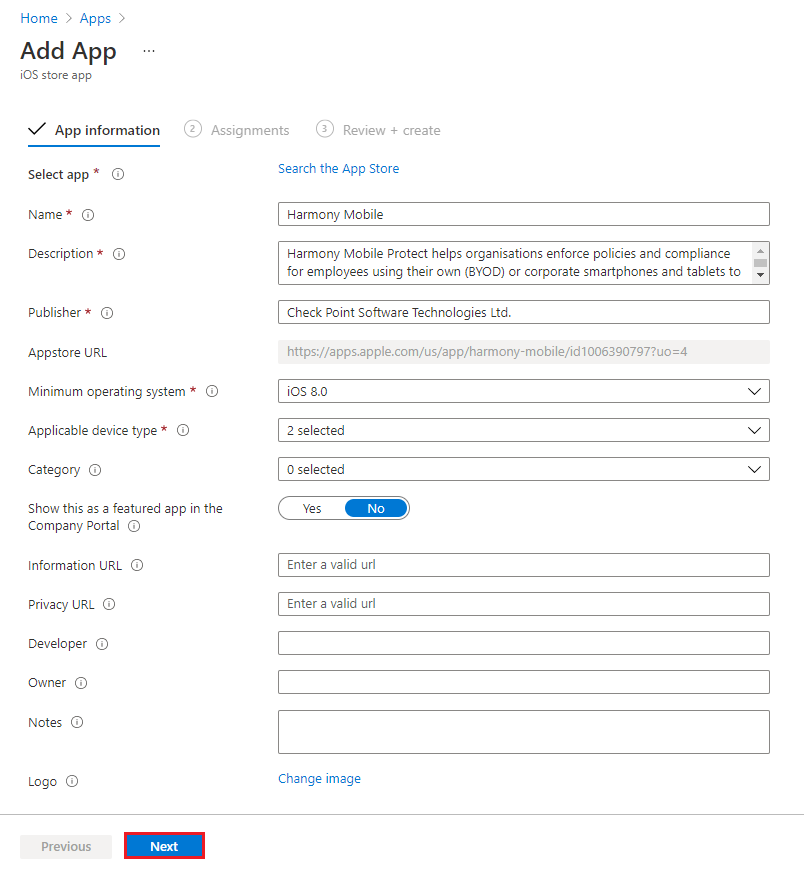This photo showcases a screenshot of a sign-up or setup page for an app, likely on a platform related to app development or management. The image is portrait-oriented and primarily features a clean, white background without any borders.

At the top, there is a breadcrumb navigation displaying "Home" in blue, followed by a right arrow, then "Apps" in blue, followed by another right arrow. Below this is a black header that reads "Add App" with a subheader "iOS Store App" in smaller text.

Further down, there are three key sections indicated for the setup process:
1. "App Information" - Marked with a black checkmark and highlighted with a blue underline.
2. "Assignments" - Denoted by a number "2" in a circle.
3. "Review and Create" - Indicated by a number "3" in a circle.

The form requires several fields to be filled out, starting with the mandatory "Select App," which is bold and black with a red asterisk, and includes a prompt to "Search the App Store." The subsequent fields include:
- **Name**
- **Description**
- **Publisher** 
- **App Store** (without an asterisk)
- **Minimum Operating System**
- **Device Type**

Additional fields without asterisks include:
- **Category**
- **Show this in Featured App**
- **Information URL**
- **Privacy URL**
- **Developer**
- **Owner**
- **Notes**
- **Logo**

Each of these options is accompanied by a rectangular white text box enabling the entry of relevant information.